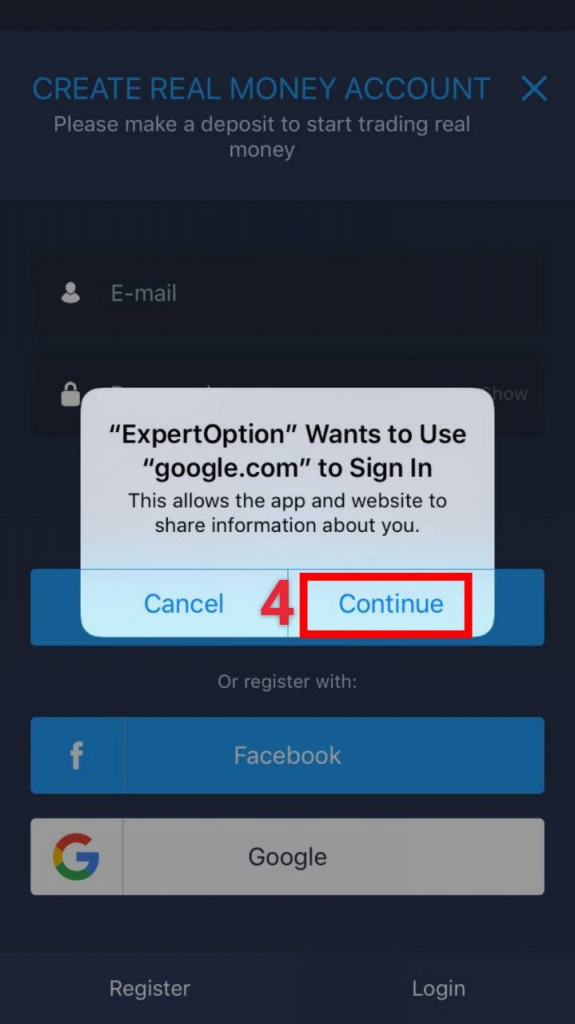This is a detailed screenshot of a user interface for a financial trading platform. The background features a gradient from a dark blue, nearly black, at the top, transitioning to a slightly lighter blue as you move down the screen. Dominating the top center is a bold, capitalized message in white: "CREATE REAL MONEY ACCOUNT." Directly underneath this text is a blue "X," followed by smaller white text that reads, "Please make a deposit to start trading real money."

Below this initial text area, the background shifts back to the darker blue. Here, a large, full-width rectangle contains the word "Email" on the left, accompanied by a small person icon. Further down, there's another large rectangle with a lock icon, but this is partially obscured by a pop-up.

The pop-up window has a white background with black text, displaying the following: 
- "Expert Option" (in quotations)
- "wants to use" followed by
- "google.com to sign in" (in quotations)

Beneath this explanatory text is a smaller line that reads, "This allows the app and website to share information about you." There are two light blue buttons at the bottom of the pop-up: the left one has dark blue text saying "Cancel," with a large red "4" between them, and the right button reads "Continue" in dark blue text, encased in a red rectangular border.

Underneath this pop-up, white text reads: "or register with." Below this line, a long blue tab stretches across the screen, displaying the word "Facebook" in white along with a Facebook icon on the left side. Just below this, there's a white rectangle with "Google" written in black, alongside the Google icon.

At the very bottom of the screen, there are two additional dark blue tabs. The left tab says "Register" in white text, while the right tab says "Log In," also in white text.